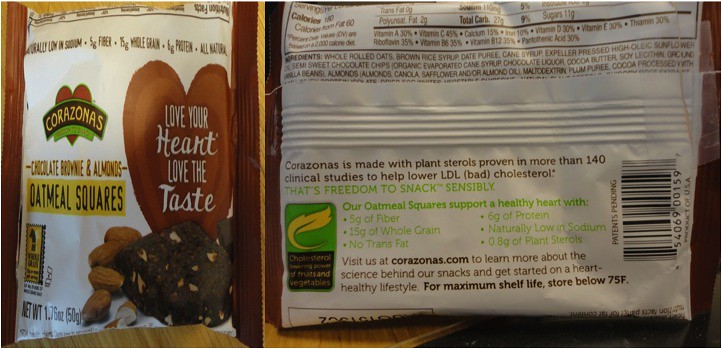The image displays the front and back views of a bag of Corazonas oatmeal squares, specifically the chocolate brownie and almond variety. The front side of the bag prominently features the Corazonas logo with a heart symbol, and the inscription “Love your heart, love the taste.” It depicts an oatmeal square that is dark brown, almost black, with visible bits of almonds surrounding a brownie, suggesting a rich, nutty flavor. 

On the left side of the bag, the packaging highlights key features such as the snack being made with whole grain oats and plant sterols, which are clinically proven to help lower LDL or "bad" cholesterol. The front also mentions that the oatmeal squares have no trans fats and are naturally low in sodium.

The back side of the bag provides detailed nutritional information: 180 calories, 60 of which are from fat, 2 grams of polyunsaturated fat, 27 grams of total carbohydrates, 5 grams of fiber, 6 grams of protein, and 0.8 grams of plant sterols. Ingredients listed include whole grain oats, whole rolled oats, brown rice syrup, date puree, semi-sweet chocolate chips, cocoa butter, soy lecithin, vanilla beans, and almonds. The back emphasizes the healthy aspects of the product, such as its 15 grams of whole grain content and the absence of trans fats. 

The packaging is predominantly white with a mix of black and green text, providing a clean and readable design. Additional information advises storing the product below 75°F for maximum shelf life and directs consumers to visit corazonas.com to learn more about heart-healthy lifestyles.